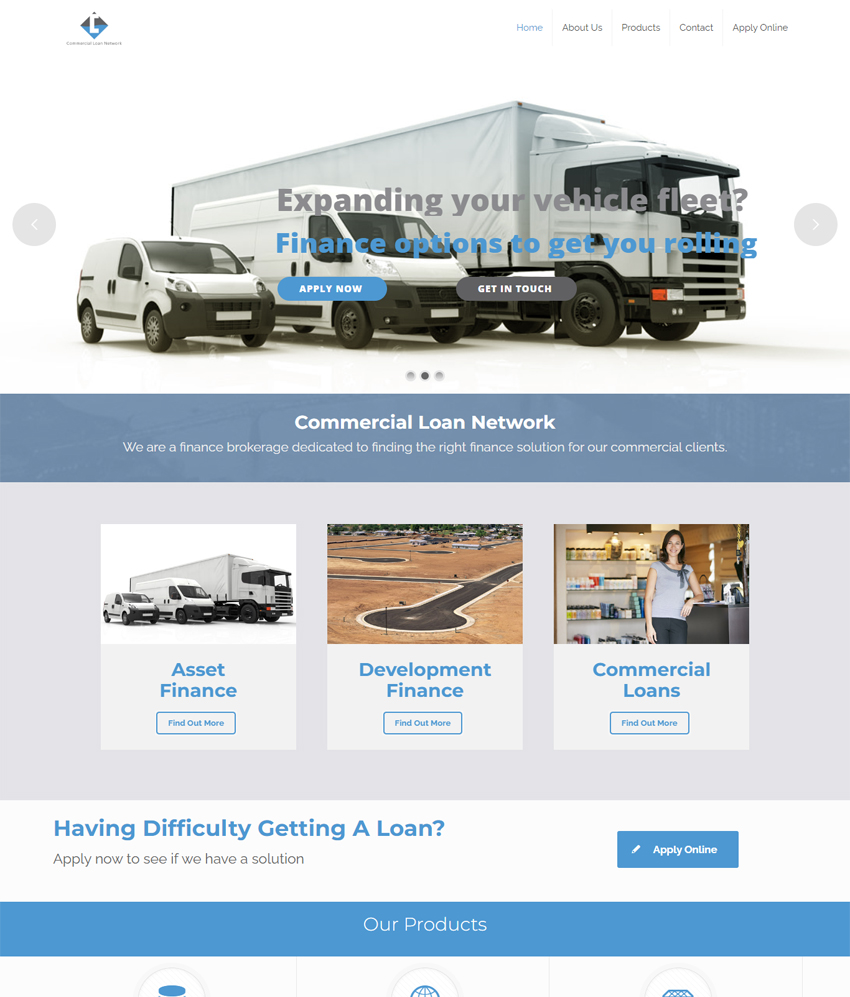This is a screenshot of a webpage detailing vehicle financing information, specifically for commercial loans. The top section features an image with a backdrop of three vehicles: a potential SUV, a larger van, and a sizable truck, all in shades of white or cream. Positioned at the top of the page is a navigation menu with five options: Home, About Us, Products, Contact, and Apply Online. In the foreground, gray text prominently reads, "Expanding Your Vehicle Fleet?" Below it, in light blue, is the phrase "Finance Options to Get You Rolling." Additionally, there is a blue pill-shaped button with white text that reads "Apply Now."